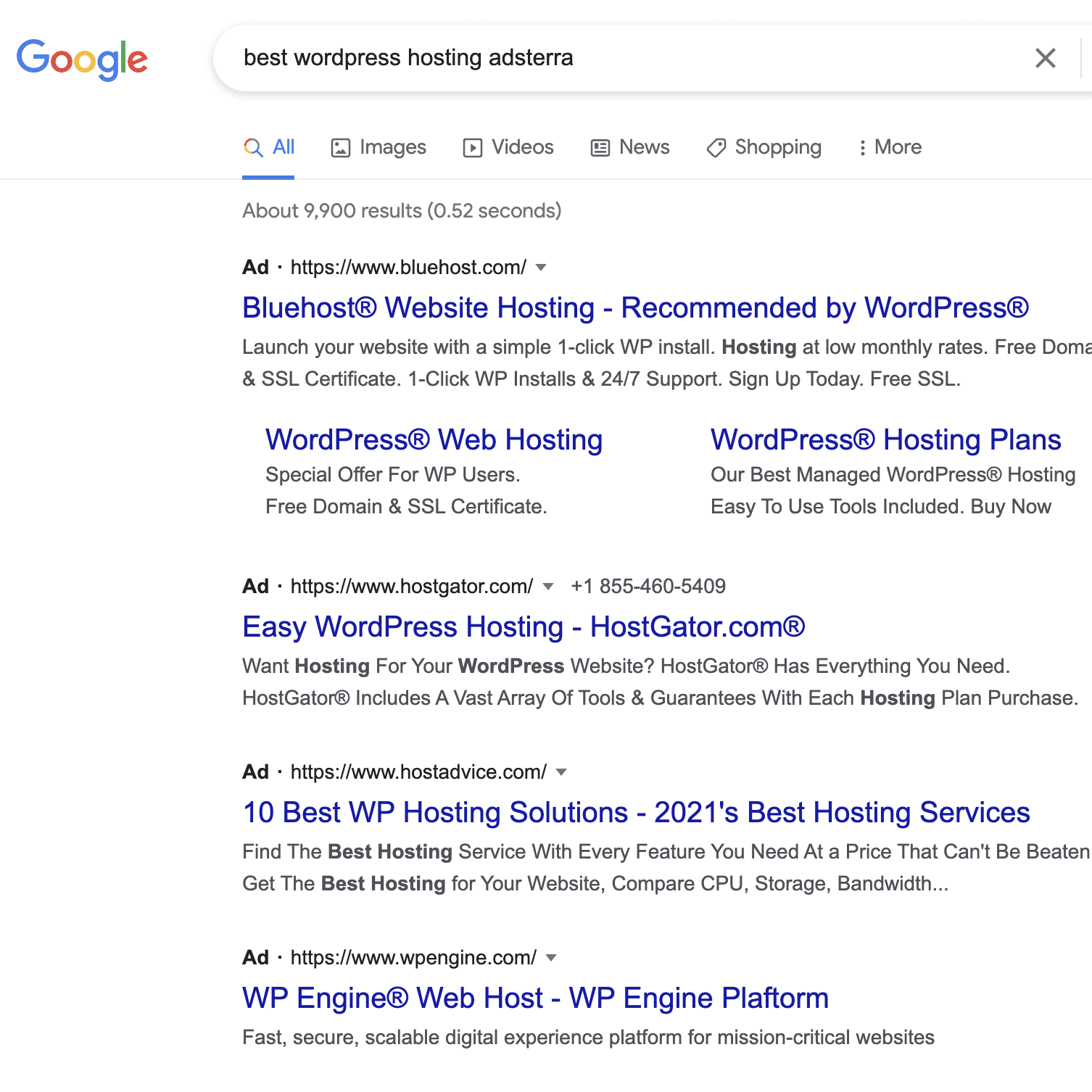A detailed caption for the provided image might read:

"The image displays a screenshot of Google search results. At the top left corner is the Google logo, while a horizontally-stretched search bar spans nearly from the center-left to the far right of the image. The search query entered is 'best WordPress hosting ad store.' Directly beneath the search bar, there are navigation tabs labeled 'All,' 'Images,' 'Videos,' 'News,' 'Shopping,' and 'More.' Immediately below these tabs, in a small font, the search results count indicates 'about 9,900 results (0.052 seconds).' The first search result is an advertisement for Bluehost.com, featuring a clickable link and a brief description. Below this, there is another advertisement for HostGator.com, also showcasing its link and description. Following this is yet another ad for HostAdvice.com, providing its link and a short description. Lastly, the final ad in view is for WP Engine, including the host link and description."